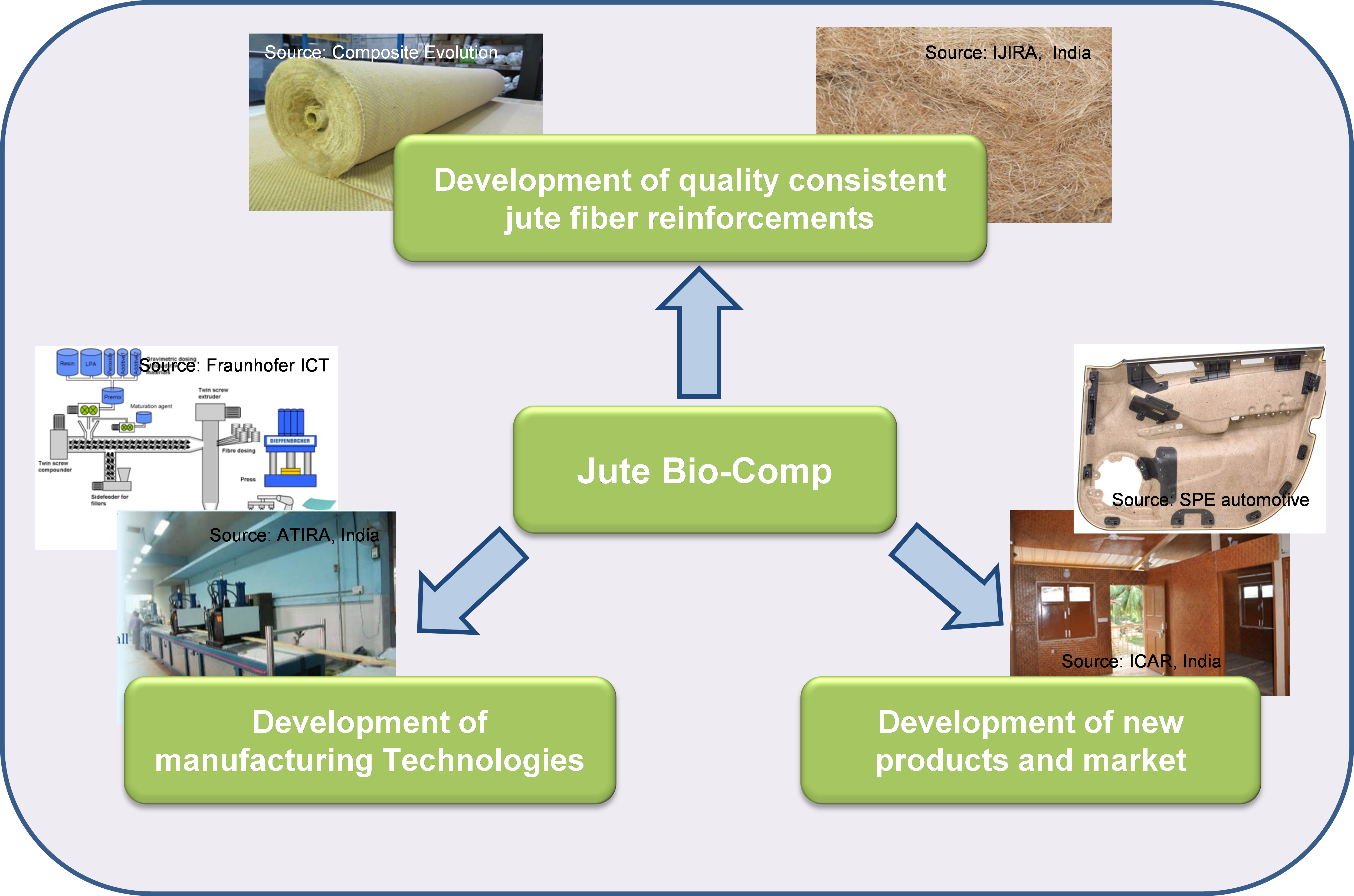The diagram features a light gray rectangular border with rounded corners and a dark gray outline, set against an off-white background. At the center is a prominent green rectangular box with white text that reads "Jute Biocomp". From this central box, three light blue arrows emerge, leading to three additional green boxes, each with white text. 

The arrow pointing upwards leads to a box labeled "Development of Quality Consistent Jute Fiber Reinforcements", flanked by two images: one of a roll of jute fibers and the other a close-up of the fibers. The downward-left arrow directs to a box labeled "Development of Manufacturing Technologies", accompanied by an image of a manufacturing facility and a diagram illustrating the manufacturing process. The downward-right arrow points to a box labeled "Development of New Products and Markets", which is illustrated by a car door panel made from jute fibers and a photo of home wall panels likely constructed from the same material.